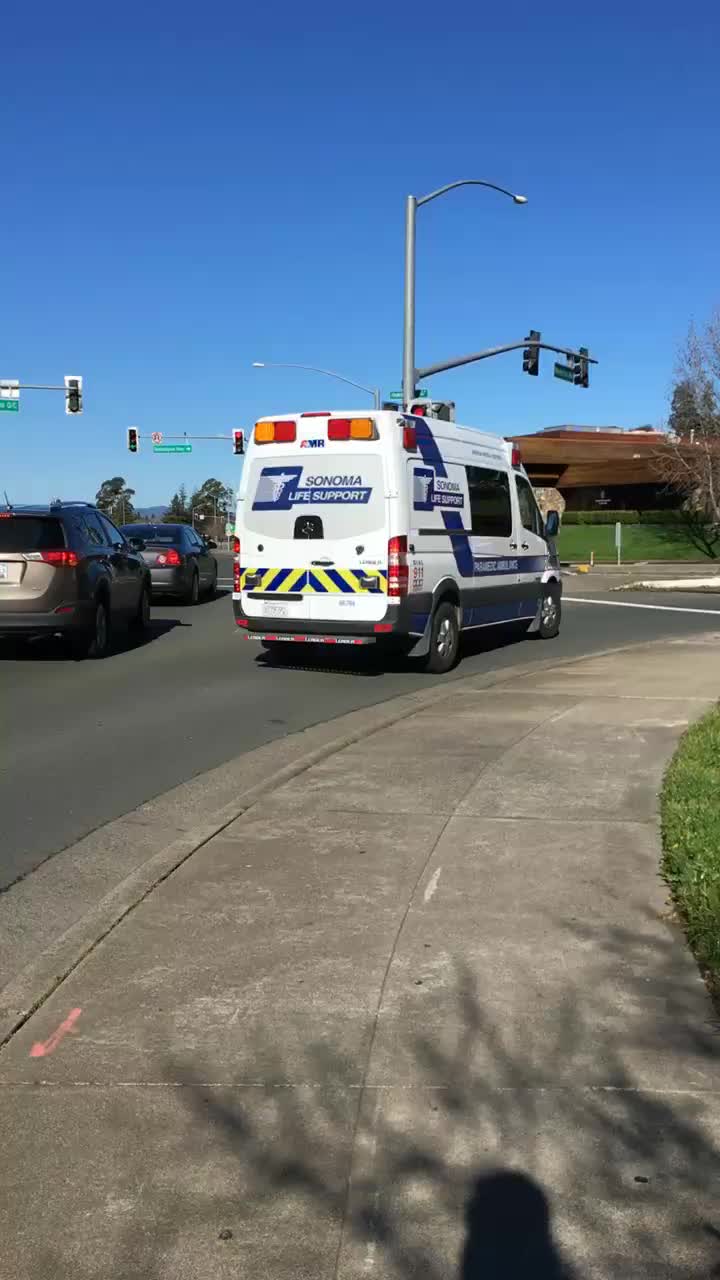In this outdoor photo, taken from the perspective of a person on a grey cement sidewalk, we see a street lined with traffic lights against a clear blue sky. In the foreground, to the right of the sidewalk, there is a green grassy area. The street itself is grey and paved, with a few cars, including an SUV and a sedan, waiting at a red light. To the right, in the right turning lane, stands a white, blue, and black ambulance with "Sonoma Life Support" in blue writing and a yellow and black sticker on the back. A traffic light pole with attached street signs and a street light rises above the scene, located near a brown brick building to the right. The combination of stopped vehicles, traffic infrastructure, and surrounding buildings suggests a typical urban intersection, with possibly commercial or office buildings in the background.